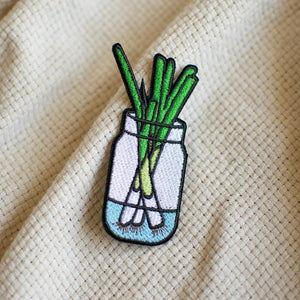This image depicts a detailed embroidered patch, likely intended as an iron-on for a shirt or t-shirt. The patch features a mason jar, outlined in black thread, partially filled with light blue water. Within the jar, three green onions are submerged root-side down, showcasing their white roots turning into light green, and then transitioning to dark green stalks emerging from the top. The waterline and jar are both bordered with black stitching for emphasis. The patch itself is positioned on a waffled, beige fabric, possibly a blanket or similar material, adding texture to the background. The jar is slightly slanted, giving the image a dynamic composition.